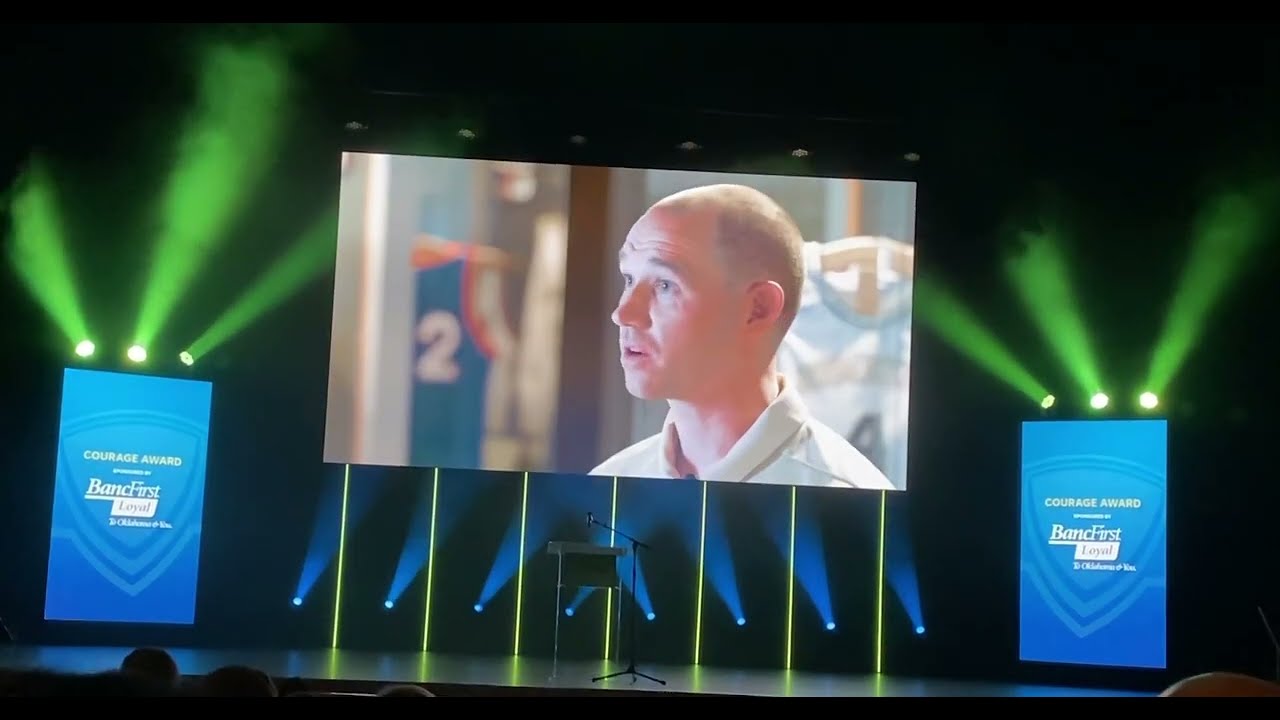The photograph captures the vibrant scene of an awards banquet stage. Dominating the background is a large central screen displaying a movie scene featuring a mostly bald Caucasian man with a surprised expression, dressed in a Miami Dolphins or Miami Heat uniform (blue with an orange outline and the white number two). Surrounding the stage, spotlights choreograph a dazzling light show: blue lights emanate from the floor, crisscrossing in both directions, while green lights, positioned about ten feet above, beam parallel shafts into the air. Additionally, green laser lights cascade down from the screen to the stage floor. On either side of the stage, two vertical rectangular screens (taller than they are wide) brandish blue backgrounds with the text "Courage Award" in white, accompanied by partially obscured text that reads something like "Bank First Level." Each of these banners is flanked by three green spotlights overhead. Centered at the forefront of the stage is a podium and a microphone stand, set against the backdrop of an audience whose silhouettes are barely discernible in the shadows. The entire setup is framed by a black background, amplifying the dramatic lighting and the sense of an intimate yet grand event.